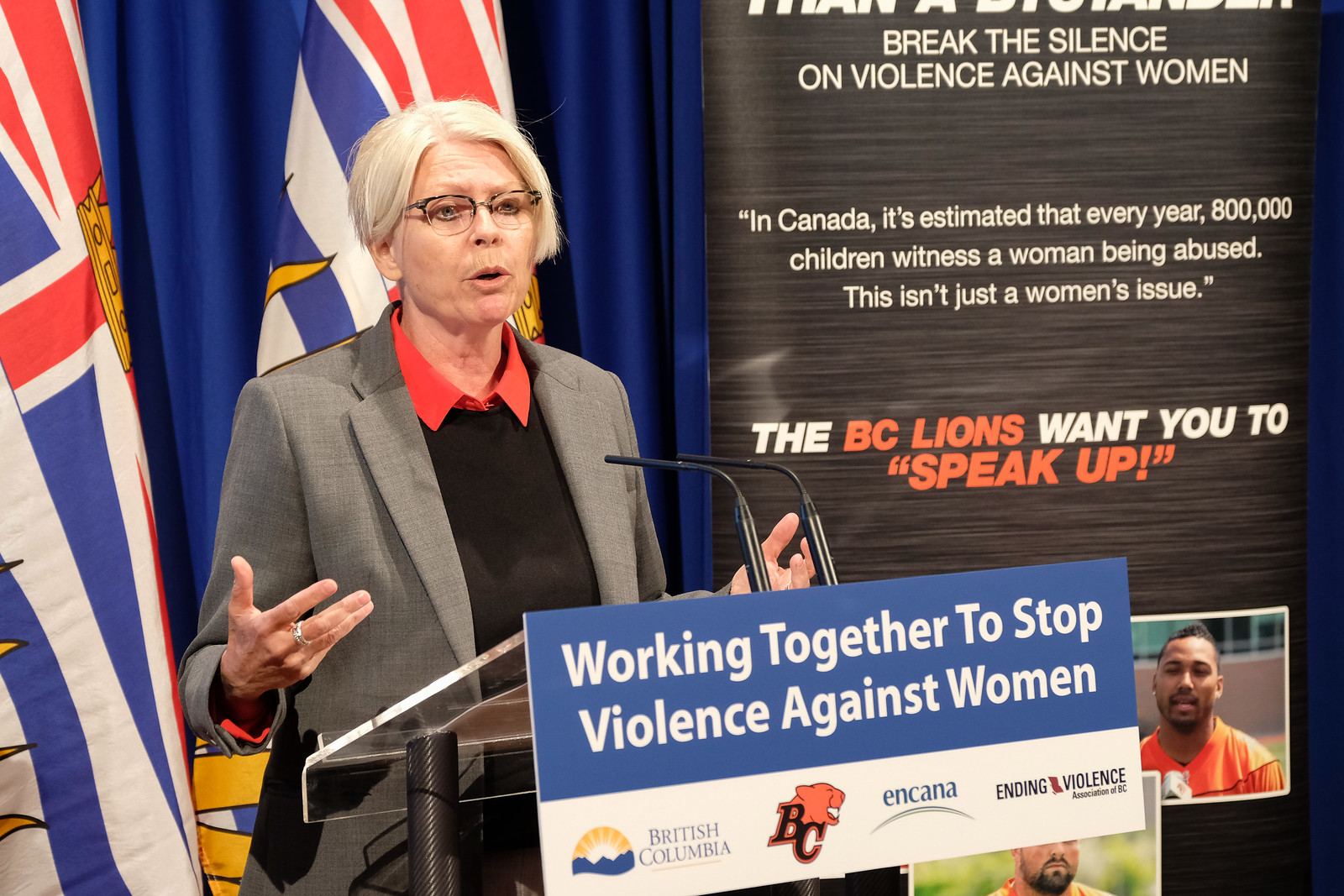The image features an older, gray-haired woman standing on a stage next to a podium, speaking passionately with her hands raised. She is wearing glasses, a red shirt beneath a black top, and a gray suit jacket. To her right, there are two microphones and two flags featuring red, blue, and white colors with crowns in the center. Behind her, a sign displays the message: "Working Together to Stop Violence Against Women," along with logos of several companies and the text "British Columbia and Canada Ending Violence in BC." There is a lion emblem also visible on the poster behind her. To her right, another sign reads: "Break the Silence on Violence Against Women. In Canada, it's estimated that every year 800,000 children witness a woman being abused. This isn't just a woman's issue." Below this text, the BC Lions' message encourages people to speak up. The poster also partially shows images of two men. The woman wears a ring on her right middle finger and stands as a strong advocate against violence in the community.